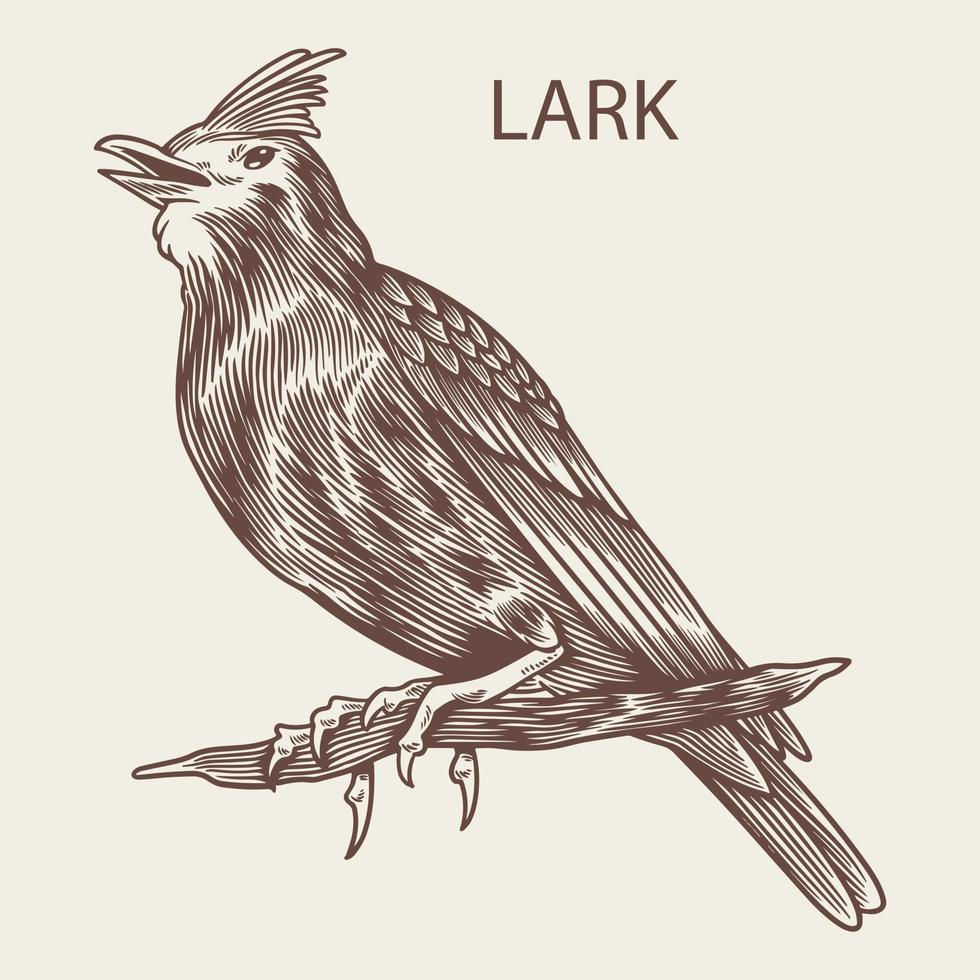The image features a detailed, line-based drawing of a bird, identified as a lark, with the word "LARK" written in plain, brown, capital letters at the top. The background is a light beige or cream color, enhancing the sepia-toned simplicity of the artwork. The bird, depicted with intricate brown lines that contour the feathers, stands on a floating segment of a branch, clasping it firmly with its sharp talons. Its mouth is slightly open and a tuft of feathers sits prominently atop its head, giving the distinct impression of a songbird in mid-chorus. The bird's elongated wings and tail are meticulously outlined, lending an air of natural elegance to its form.